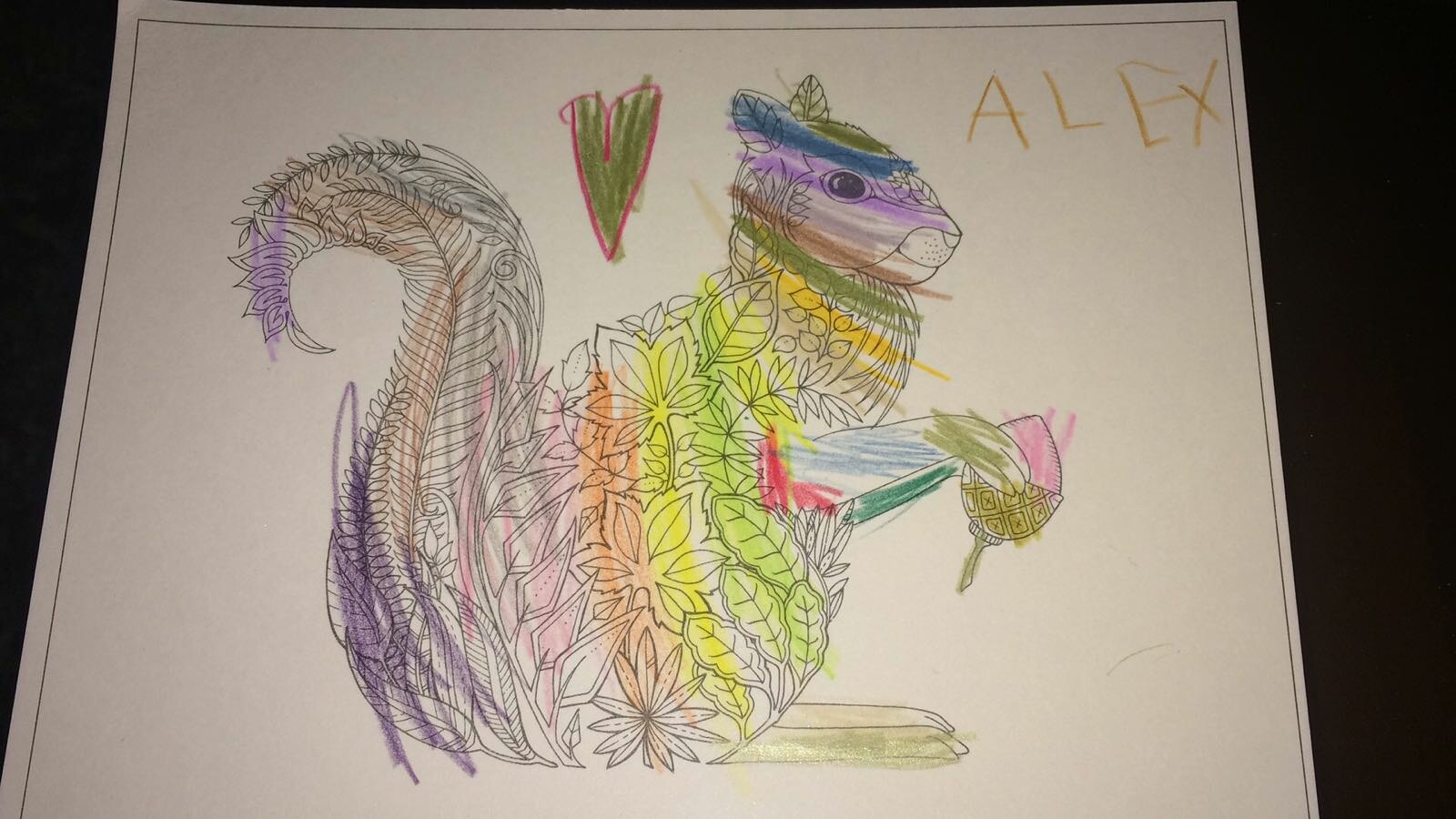This is a photograph of a child's coloring book page set against a black background. The page features a squirrel holding an acorn, with its body and tail composed of individual leaf designs. Colored mostly with crayon, the artwork displays a vibrant mishmash of hues including purple, brown, pink, orange, yellow, green, red, dark yellow, dark green, dark purple, light purple, and blue. The coloring is done in a scribbled manner, characteristic of a child's playful and carefree approach, often coloring outside the lines. At the top center of the page, a red outlined heart is filled with dark green crayon. In the top right corner, "ALEX" is written in yellow crayon, likely by the child artist, adding a personalized touch to the piece. The overall scene captures the innocence and creativity of a child's artwork, framed by a simple black square.